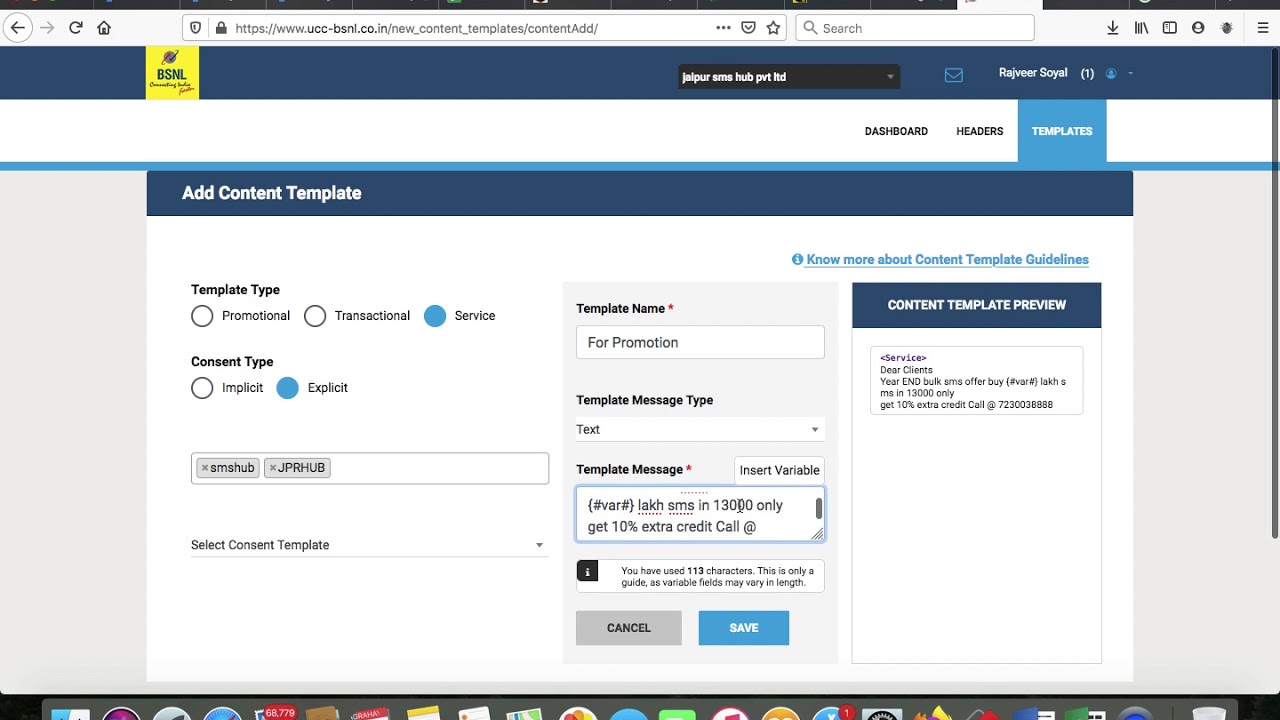Screenshot of a website interface for creating and managing content templates. The page features a black background with a continuous row of half-visible MacBook or Linux icons at the bottom. The text is quite small and detailed. At the top, the URL displayed is "www.ucc.co.in/new_content_templates/content/add." A search box is present alongside a blue band on the left, adjacent to a yellow square with "BSNL" written on it, followed by an image of a planet with a ring around it. Below this is a black box labeled "Jaloper SMS Hub PXT Limited," which is a pull-down menu, alongside a mail icon and the name "Rajveer Sohail" with one notification.

A white band below this displays several sections. On the right side, dashboard headers and templates are selected in blue. Below it, there is a band labeled "Add Content Template." This section includes options such as template types, with "Promotional" and "Transactional Services" highlighted in blue, and content type "Implicit" and "Explicit" selected. Two tags, "SMS Hub JP" or "Hub," appear underneath.

Further down is a field for entering the template name and template message type, with text boxes for the template message. The message reads, "Get an extra 10% credit call at..." with HTML characters interspersed. A note beneath states, "You've used 113 characters; this is only a guide, as variable feeds may vary in length."

At the bottom are a grey "Cancel" button and a blue "Save" button. To the right, another blue button labeled "Content Template Preview" allows clients to preview the message text. There is also a note on bulk SMS offers: "Your end bulk SMS offer by VAR lacks MS in 13,000 only, get 10 extra credit call, long number." At the top of this section, a hyperlink to "Know more about content template guidelines" is available in blue.